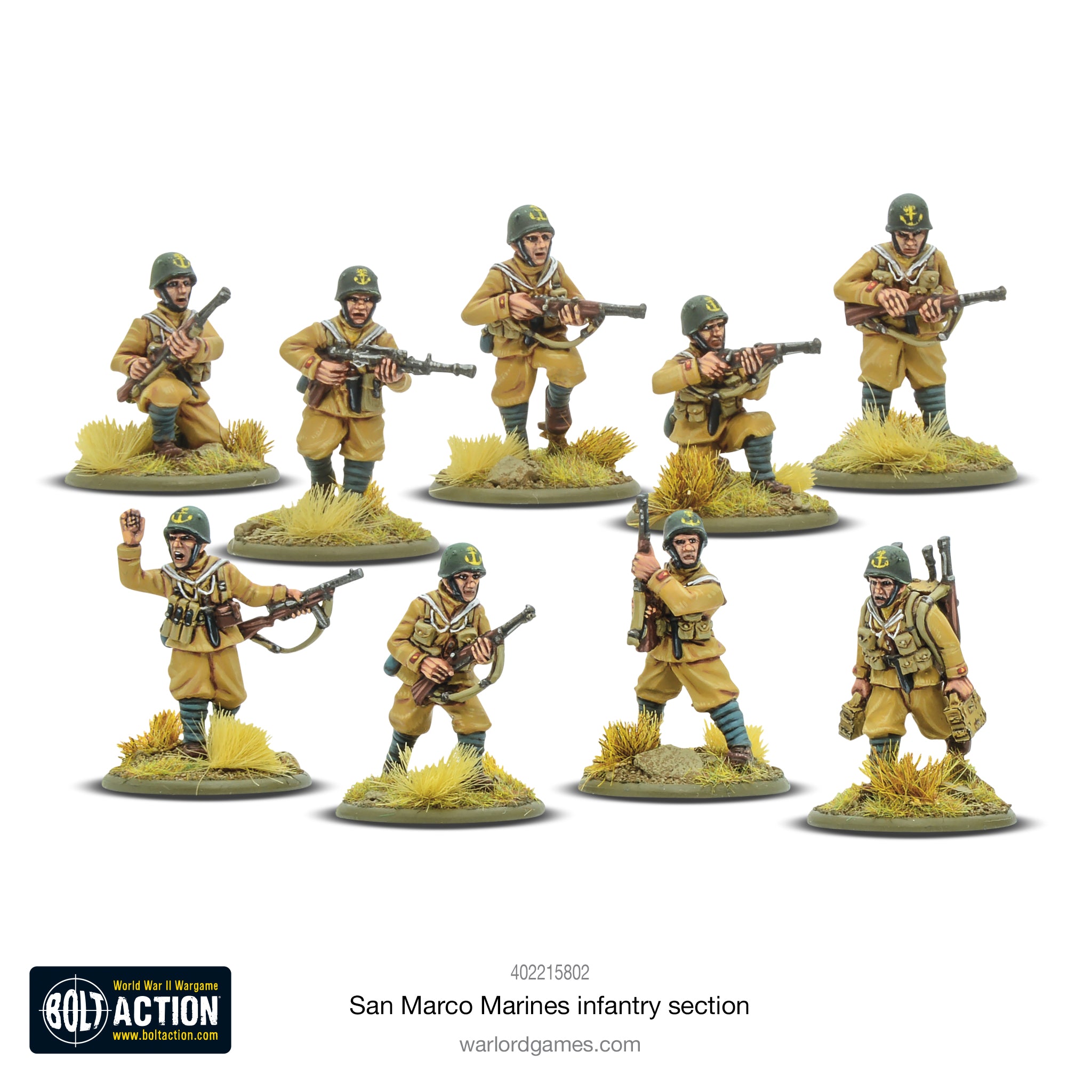The image showcases a detailed collection of nine miniature San Marco Marines Infantry Section figures by Warlord Games. Each marine is uniquely posed and connected to a round, green base adorned with 3D rocks and tufts of grass. The soldiers are attired in khaki uniforms, and their stances vary from kneeling and aiming, to standing and holding rifles. One figure is depicted walking with a gun strapped to his back, carrying blocks, while another appears to be waving. The meticulous craftsmanship and the variety of poses elicit the realistic semblance of a World War-themed tabletop wargame. Towards the bottom of the image, the text reads "San Marco Marines Infantry Section," "WarlordGames.com," and "BoltAction.com," signing off with the logos of these websites.